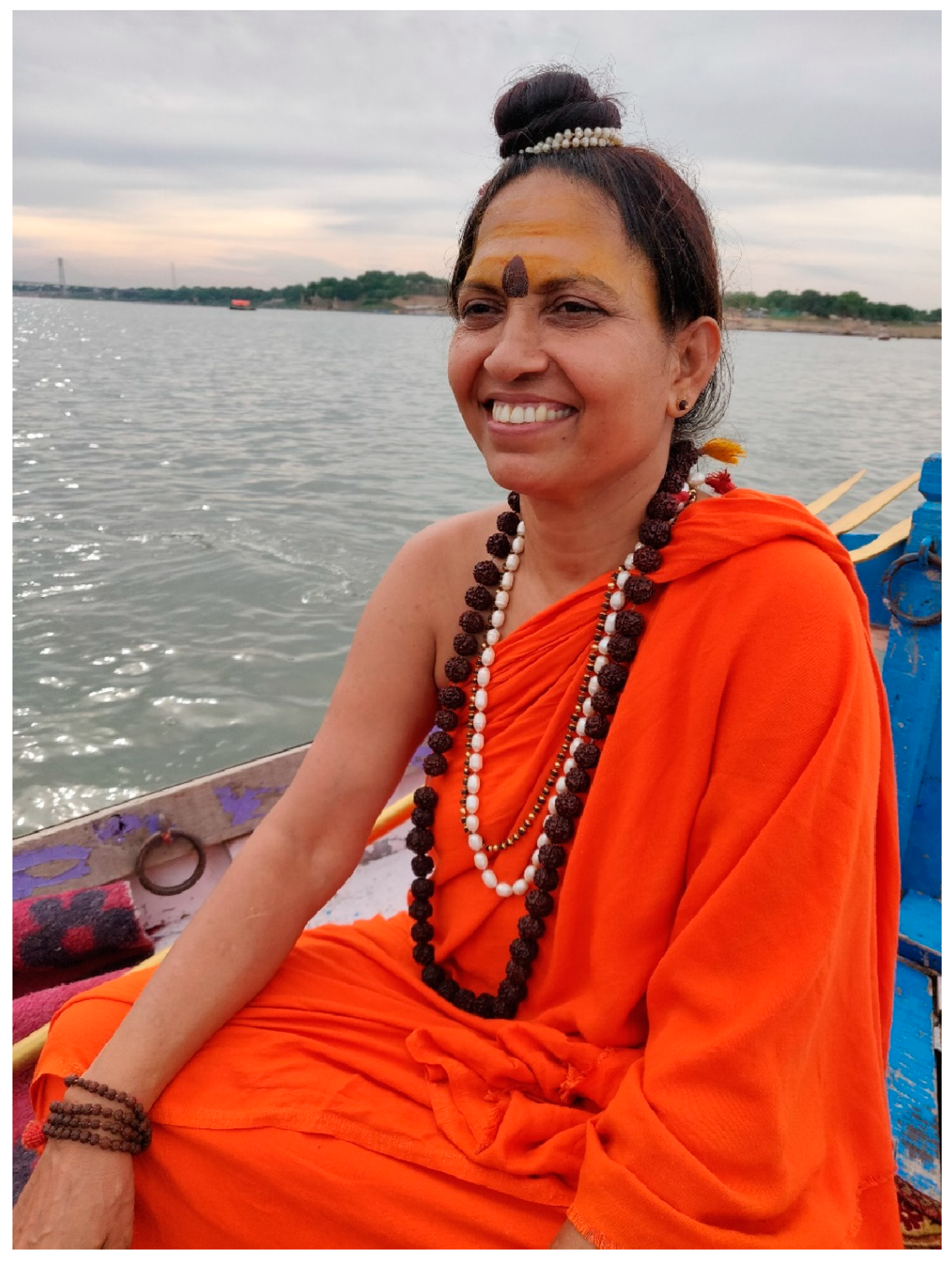In the image, a smiling woman is seated in a small, blue boat that floats on a vast body of rippling water. She dons a bright orange robe that drapes over one shoulder, resembling traditional Buddhist attire. Her hair is styled in a top knot bun adorned with a white beaded cord. Around her neck, she wears three distinct bead necklaces: one with large, dark brown beads, another with white beads, and a third with smaller, golden beads. Her wrist is decorated with a brown beaded bracelet, and she has small earrings. Her forehead is painted with a yellowish streak, accompanied by a striking black pear-shaped dot between her eyebrows. The woman exudes a sense of calm and joy as she looks to the left, and distant land is visible behind her on the horizon.